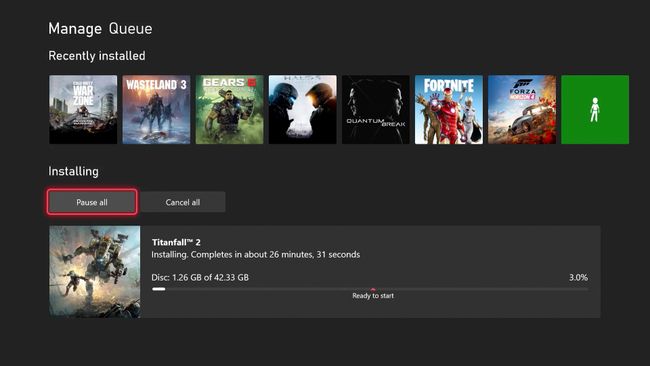The webpage features a sleek black background with the title "Manage Q" prominently displayed in the upper left corner. Below the title, two main sections organize content related to game installations. 

The first section, labeled "Recently Installed," showcases a horizontal list of eight album covers, each representing different games. These covers are accompanied by titles and images, some depicting people in various scenarios. The games listed here include Warzone, Wasteland 3, Gears, a game featuring two people wearing helmets, Quantum Dream with a striking black silhouette, the ever-popular Fortnite, Forza with a distinctive green background, and a game identifiable by a white silhouette on a green background.

The second section, titled "Installing," details the progress of ongoing installations. Here, you have options to either "Pause All" or "Cancel All," with "Pause All" already selected and highlighted in red. One specific installation shown is Titanfall 2, which is 3% completed, indicating that 1.2 gigabytes of the total 42.3 gigabytes have been installed. The estimated time for completion is 26 minutes and 31 seconds. Users can choose to unpause or cancel the installation through options on the right-hand side of the screen.

Overall, this webpage is a well-organized and user-friendly interface for managing game installations, featuring clear sections for recent completions and ongoing processes.